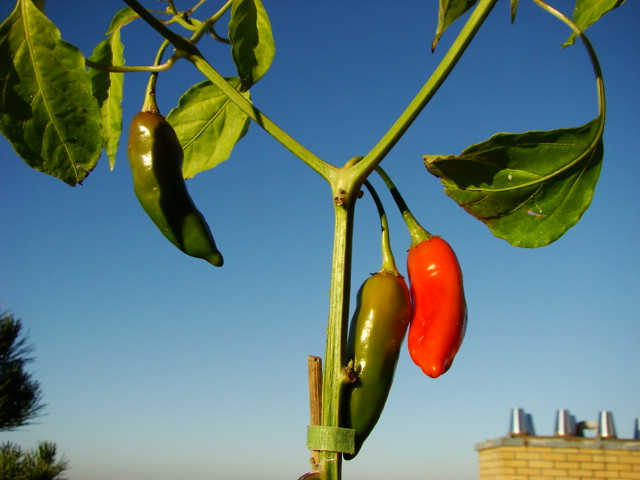This slightly out-of-focus color snapshot captures a vibrant pepper plant, believed to be a jalapeño, as its central subject. The plant's green stalk, bound with a green tape to a wooden stake at the bottom center, rises gracefully before splitting into a Y-shaped formation. From this central fork, three peppers dangle: one fully matured to a striking red, and two other predominantly green peppers with hints of red starting to appear. The foliage is marked with green leaves that glisten under the sun, each leaf showing textured markings. The backdrop features a brilliant, clear blue sky, with a portion of a tree's brush creeping into the lower left corner of the frame. On the bottom left side, a brick building with a metal decoration, resembling a chimney with tan bricks and capped with gray stone, adds a touch of urban context to the image. The scene suggests the possibility of a rooftop garden, juxtaposing nature with the hint of an architectural element.